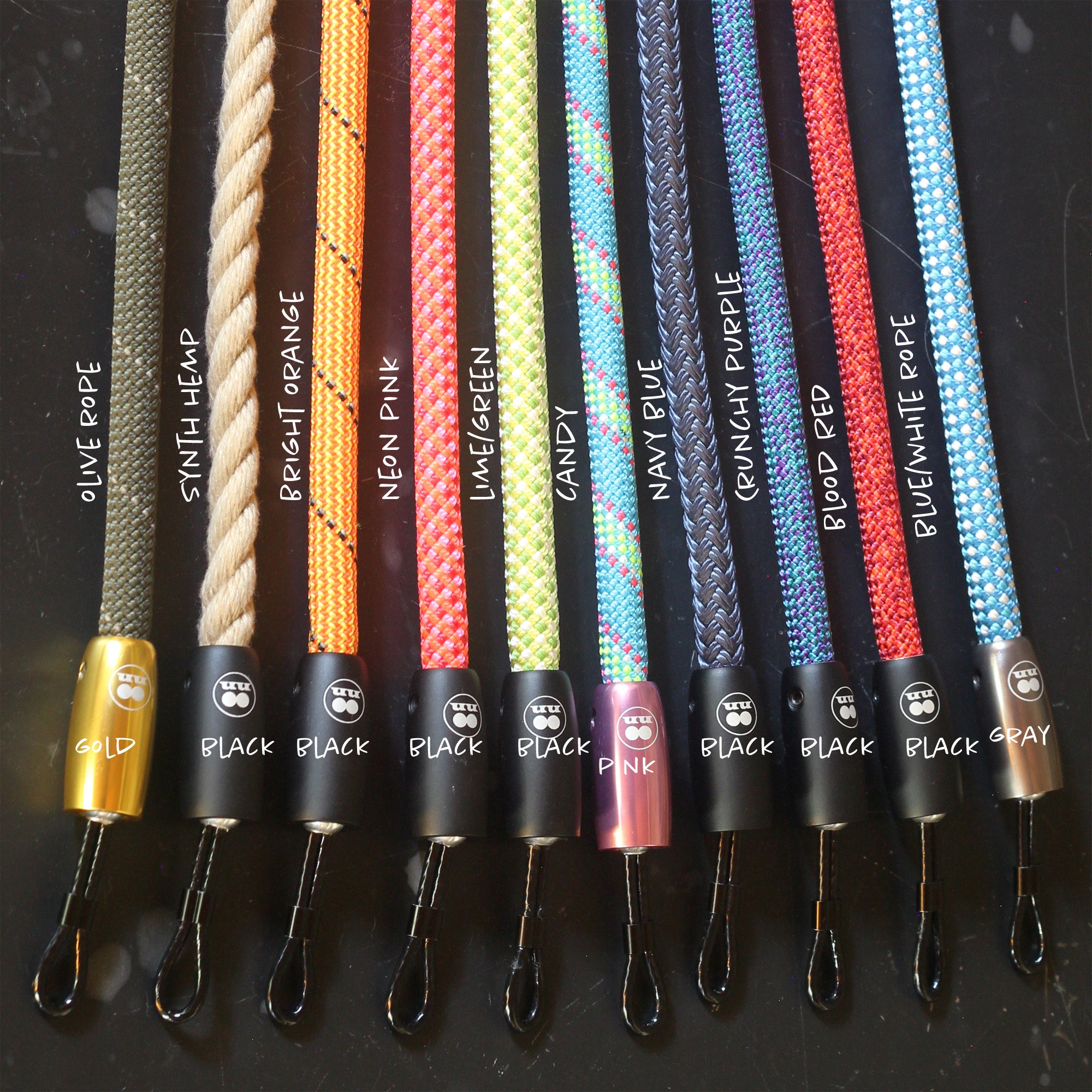The image showcases a collection of colorful, woven camera straps neatly laid out side by side on a black background. Each strap, made from various materials such as olive rope, synthetic hemp, and blue-white rope, displays a wide range of vibrant colors including bright orange, neon pink, lime green, candy, navy blue, raunchy purple, and blood red. The ends of the straps feature metal clasps in a variety of finishes—black, gold, pink, and gray—with imprinted logos and swivel clips attached for added functionality. Text next to each strap highlights both the color and material used, suggesting that this is a display likely intended for a store, showcasing the diverse options available to customers. The straps are intricately woven and thick, indicating their durability, possibly suitable for rugged use such as climbing.